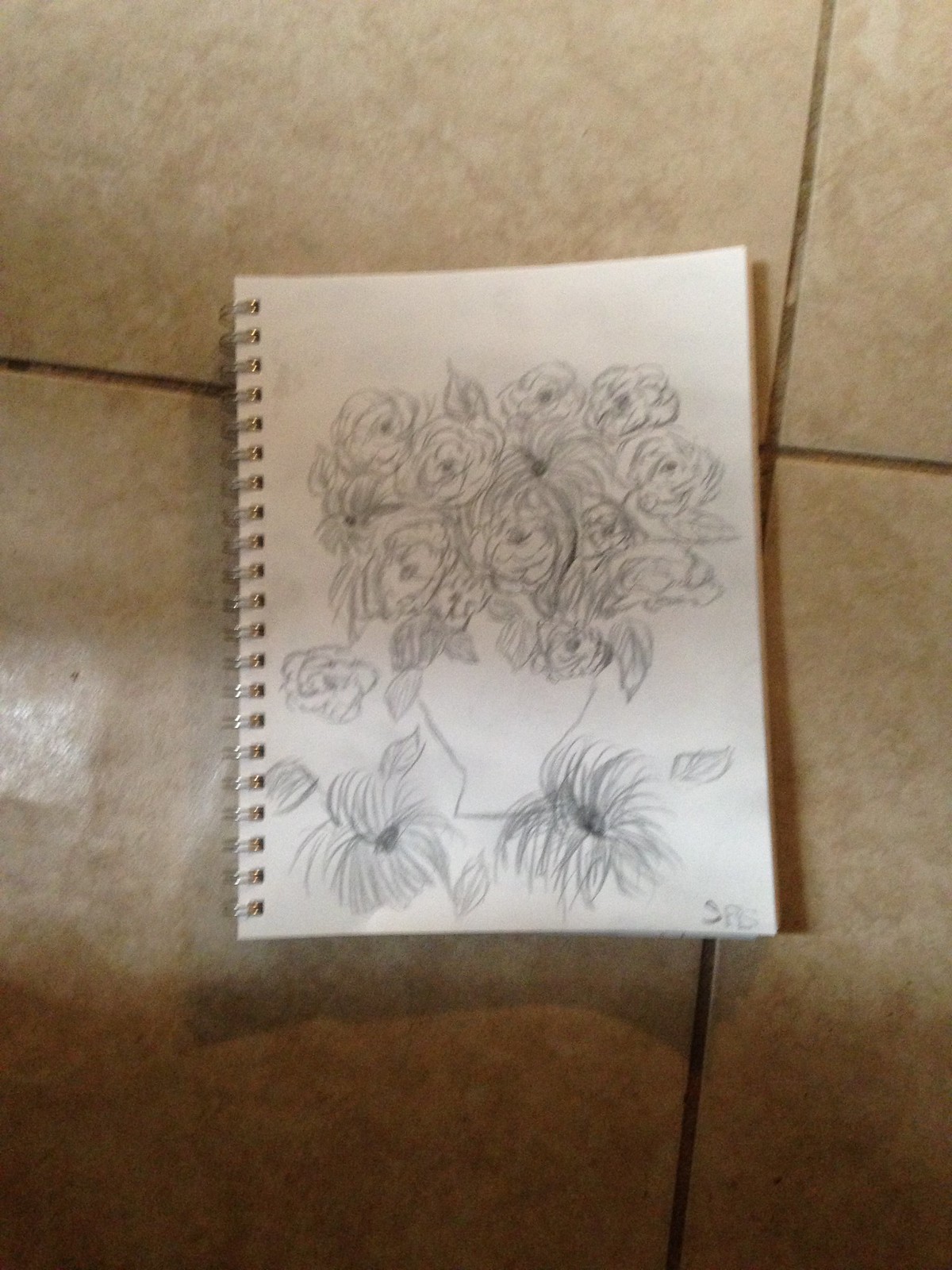This image captures a color photograph taken inside a room, featuring a binder-type sketchbook lying on a polished, brown-tiled floor. The image is slightly tilted to the left by about 10-15 degrees. The tiles have visible brown grout and reflect light in the middle left of the photograph. 

At the center of the image is the open sketchbook, turned to a white page displaying a detailed black and white drawing. The sketch, executed in pencil or black ink, depicts a vase that flares out towards the top. The vase is filled with an abundant bouquet of highly detailed flowers, likely roses, with individually shaded petals and leaves. Surrounding the vase on the page are three smaller, peculiar-looking flowers, possibly preliminary sketches or practice drawings. The bottom right of the page contains a signature, "SRS." The polished tiles and the carefully detailed sketches contribute to the sense of precision and artistic endeavor captured in the photo.